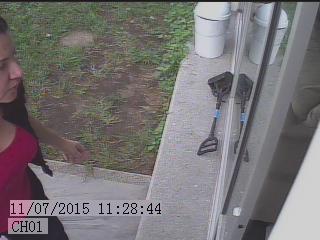The image, a small, blurry square likely taken from a CCTV camera, captures a moment in time on 11/07/2015 at 11:28:44, as indicated in the lower left-hand corner along with the label "CH01." In the frame, a young woman with long brown hair, dressed in a form-fitting, low-cut red top and black pants, appears on the far left-hand side, walking towards the right. She seems to be approaching a stone gray ledge with the intention of picking something up. The ledge holds a small white container or bucket and a black object resembling a dog pooper scooper. On the right side of the image, there is a glass sliding door, through which the white container and cleaning tools can be seen reflected. The upper left-hand side of the picture shows some dirt and grass, suggesting an outdoor or semi-outdoor setting. The woman occupies about 10% of the frame as she moves towards the entrance near the door.